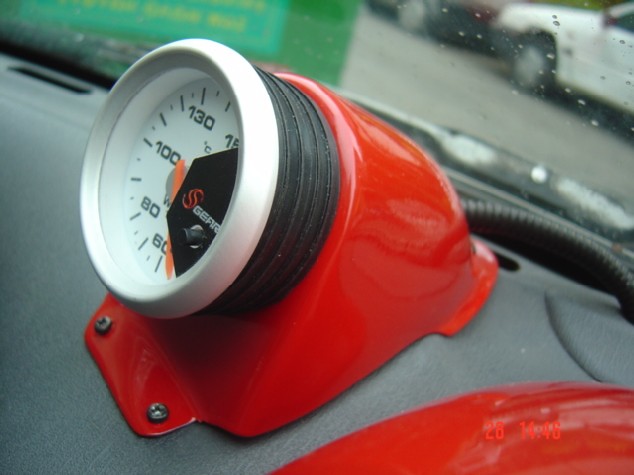The image captures the interior of a car, prominently showcasing the front dashboard. Through the rain-speckled windshield, droplets are visible along with windshield wipers in their idle position. Outside, a white car is either parked or following directly behind a reddish-maroon vehicle, with both cars' tires visible. Ahead, there's a green object, possibly the rear of a truck or a large container, identifiable by its square shape.

On the dashboard, there's a prominently featured red base mount holding a circular, black-rimmed device with a white face displaying measurements, which seems to be an aftermarket speedometer. The speedometer features a white background with gray numbers and lines marking the increments, accompanied by an orange needle. The brand name "Gephri" is printed on the device. Additional elements on the dashboard include a shiny red object and a black tubing running along the windshield’s edge.